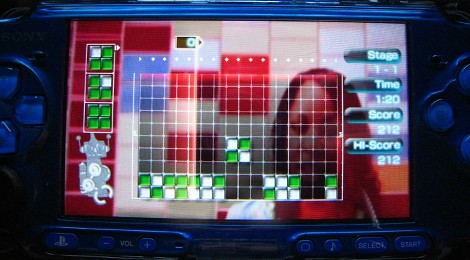In this nighttime image, we are presented with the intricate view of a car dashboard. Dominating the scene is a large, rectangular, illuminated screen that seems designed for navigation, stretching from left to right. To the left of this screen, partially visible, is a small, black steering wheel. The background is entirely black, enhancing the luminous elements on the display. 

On the screen, at center right, is an overlaid image of a female head with dark hair, her facial features indistinguishable. Superimposed over her head, there is a graphical representation consisting of white lines forming a grid-like pattern, with small boxes within the grid checked in green and white. To the left of these boxes, more green squares can be seen. 

From the upper right corner of the screen, descending, the following information is displayed: "Stage 1 to 1," "Time 1 minute 20," "Score 212," and "High score 212." Beneath the screen, the dashboard's control buttons reside, blending into the black background. At the lower right corner, there are buttons labeled "Select" and "Start." On the lower left, volume control buttons labeled "Volume -" and "Volume +" are visible.